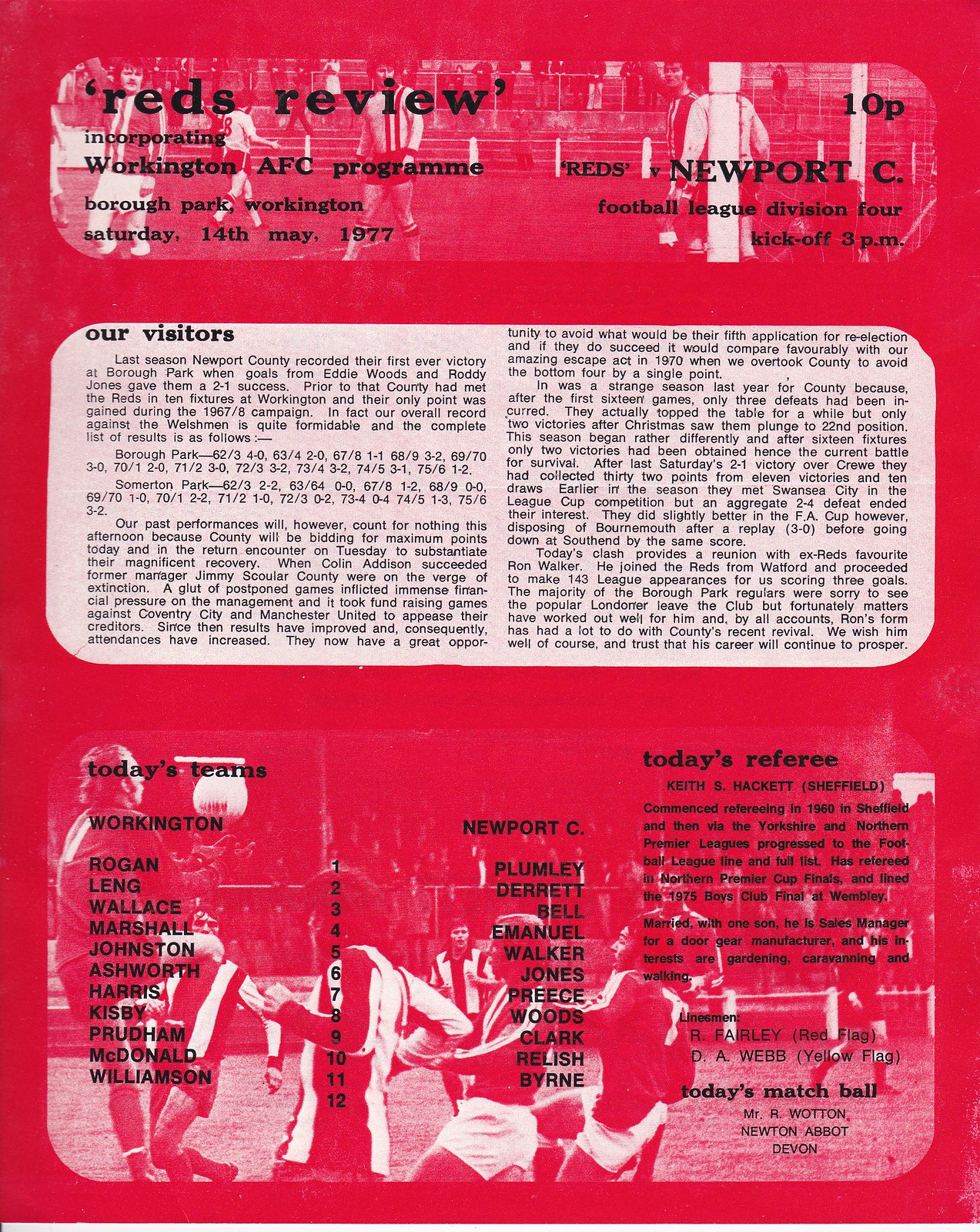The image displays a detailed, digitally-rendered poster with a prominent red background, divided into three main sections. At the top left, in bold black text, it features the title "Reds Review," with a subheading that reads, "Incorporating Workington AFC Program, Borough Park, Workington, Saturday, 14th May 1977." The price noted is 10p and the event details specify, "Reds vs Newport C, Football League Division 4, kick-off 3pm."

Beneath this, a white box with black text highlights the section titled "Our Visitors." This section reviews Newport County's football history at Borough Park, noting their first-ever victory there last season with a 2-1 success attributed to goals from Eddie Woods and Roddy Jones. It also mentions previous encounters, indicating that Newport County had only earned a single point at Workington, during the 1967 campaign.

At the bottom of the poster, the section is divided into two columns under the heading "Today's Teams." It lists the players for both Workington and Newport County. Workington's lineup includes Rogan, Lang, Wallace, Marshall, Johnston, Ashworth, Harris, Kisbee, Prudham, McDonald, and Williamson. Newport County's lineup features Plumlee, Derrett, Bell, Emmanuel, Walker, Jones, Preece, Woods, Clark, Relish, and Brine. Additionally, this section specifies that today's referee is Keith S. Hackett of Sheffield, accompanied by information about the match officials and the match ball.